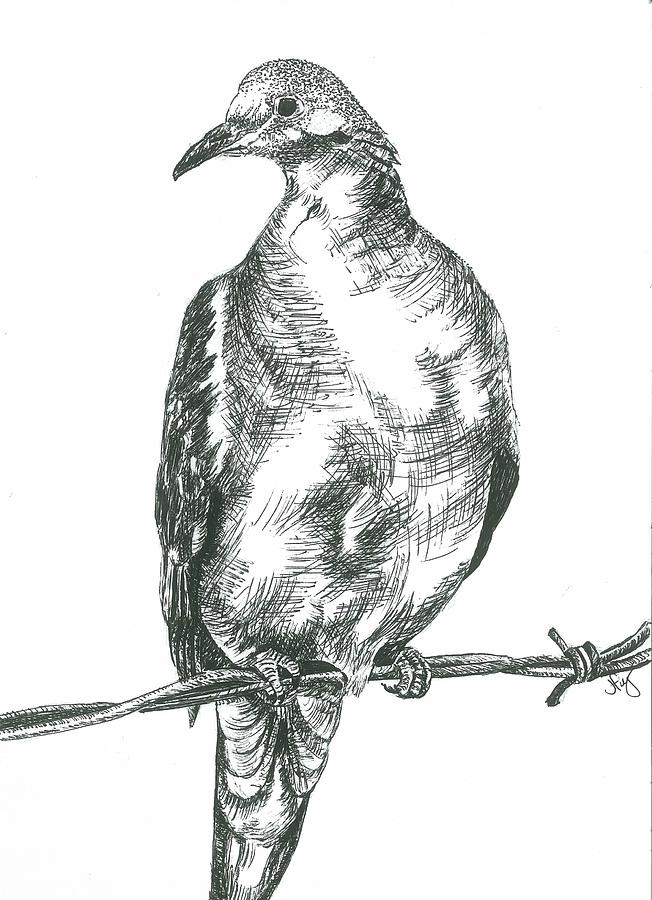This highly detailed, grayscale illustration depicts a bird perched on a slender, twisty branch. The monochromatic palette utilizes dark gray and white tones to create a visually striking image. The bird's claws are meticulously wrapped around the branch, while a thin piece of twine or rope appears to be tied around one end of the branch beneath the bird. 

With one eye visible, the bird gazes off to the side, and its dark beak contrasts sharply against the lighter tones. The craftsmanship of the illustration is evident in the individual, pencil-like markings that define the feathers. Toward the head, sparse white patches add texture and depth, enhancing the intricate detailing of the feathers and tail. 

An artist's signature, subtle and small, sits quietly under the branch, contributing to the authenticity and completeness of this elaborate drawing. The image boasts crystal clear quality, making the elaborate tail feathers and feather details on the head stand out vividly.